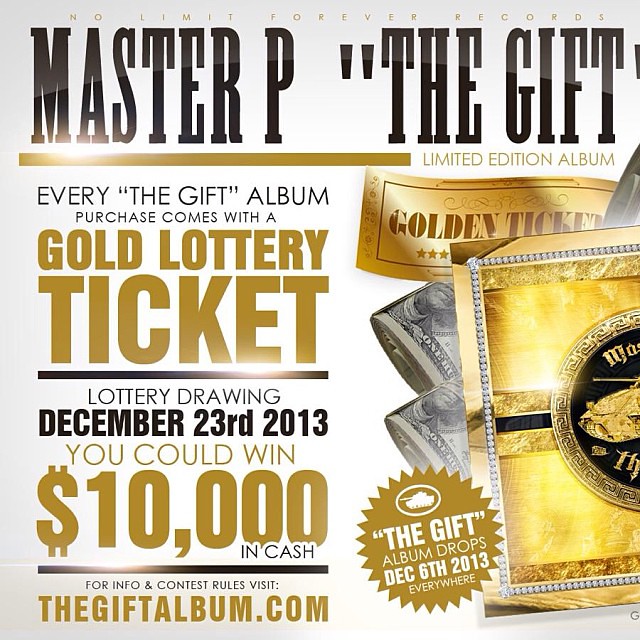The image appears to be an advertisement for Master P's "The Gift" Limited Edition Album, released by No Limit Forever Records. At the top, it prominently displays the text "No Limit Forever Records" in gold, and "Master P The Gift" in bold black font. The advertisement highlights that every purchase of "The Gift" album includes a gold lottery ticket, with a drawing set for December 23, 2013, where the winner could receive $10,000 in cash. For detailed information and contest rules, it directs viewers to visit thegiftalbum.com.

On the right side of the image, there is a depiction of a gold album, presumably the cover of "The Gift," surrounded by rolls of $100 bills, enhancing the luxurious theme. A golden ticket, reminiscent of those from "Charlie and the Chocolate Factory," is also featured prominently. The advertisement additionally includes a circular sunburst design at the bottom, partly covering the money and gold items. A badge within this design states that "The Gift" album will be available everywhere starting December 6, 2013.

The color scheme predominantly features gold and black, with green hues from the dollar bills and a white background, aligning with the high-end and exclusive feel of the promotion.